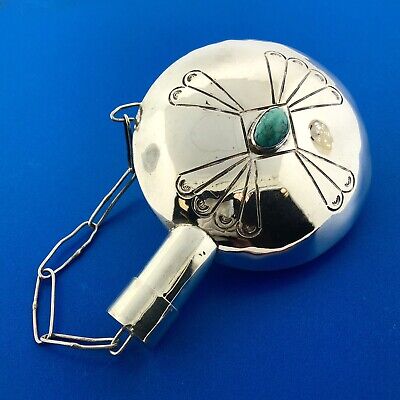The image captures a finely detailed silver pendant set against a rich royal blue background. The pendant, highly polished and disc-shaped, is attached to a silver chain that extends to the left. Centrally featured is an embedded turquoise stone, oval in shape, surrounded by an etched triangular pattern. Radiating from this center are intricate feather-like etchings, forming a cross shape with four segments at the top and bottom, and two segments on either side. The pendant, reminiscent of a pocket watch in its design, also includes a tubular piece at the bottom where the chain connects.